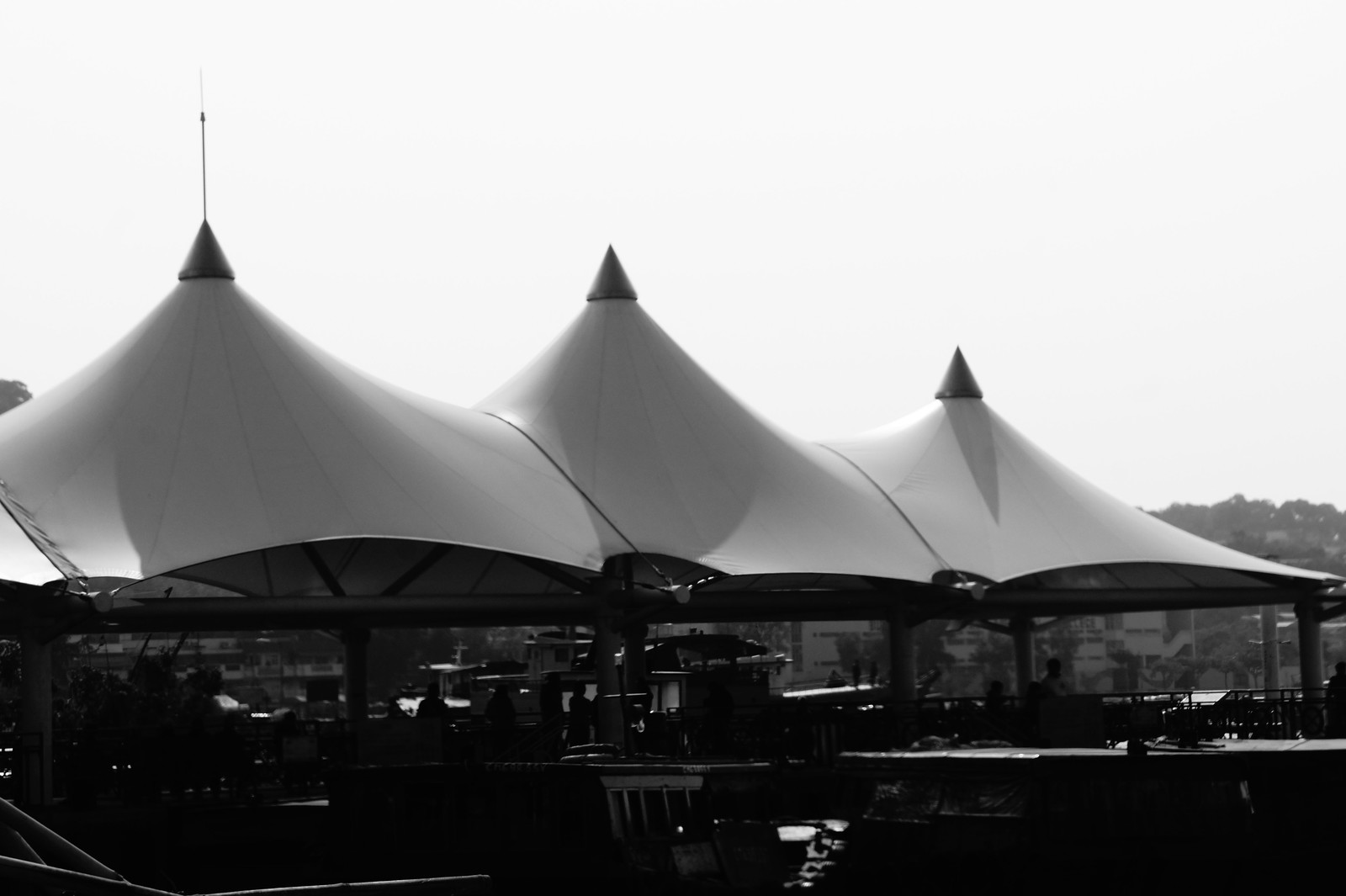This black-and-white photograph captures a man-made outdoor sitting area featuring three distinctive tent-like structures with pointed, black-tipped tops. The pavilions create a shaded space, giving the appearance of sophisticated, steeple-like roofs, one of which is adorned with an antenna. Despite the black-and-white format, there is a suggestion of coloration, hinting at a possibly red hue. The scene, darkly lit, makes it difficult to discern specific details within the shaded area, which includes chairs, tables, and indistinct outlines of people. The setting appears to be a fancy dock or waterfront facility, with a boat visible in the background and a white building with unusually shaped windows on the far right. The photograph captures shadowed trees at the left corner and the far right distance, contrasting with the stark white sky above.